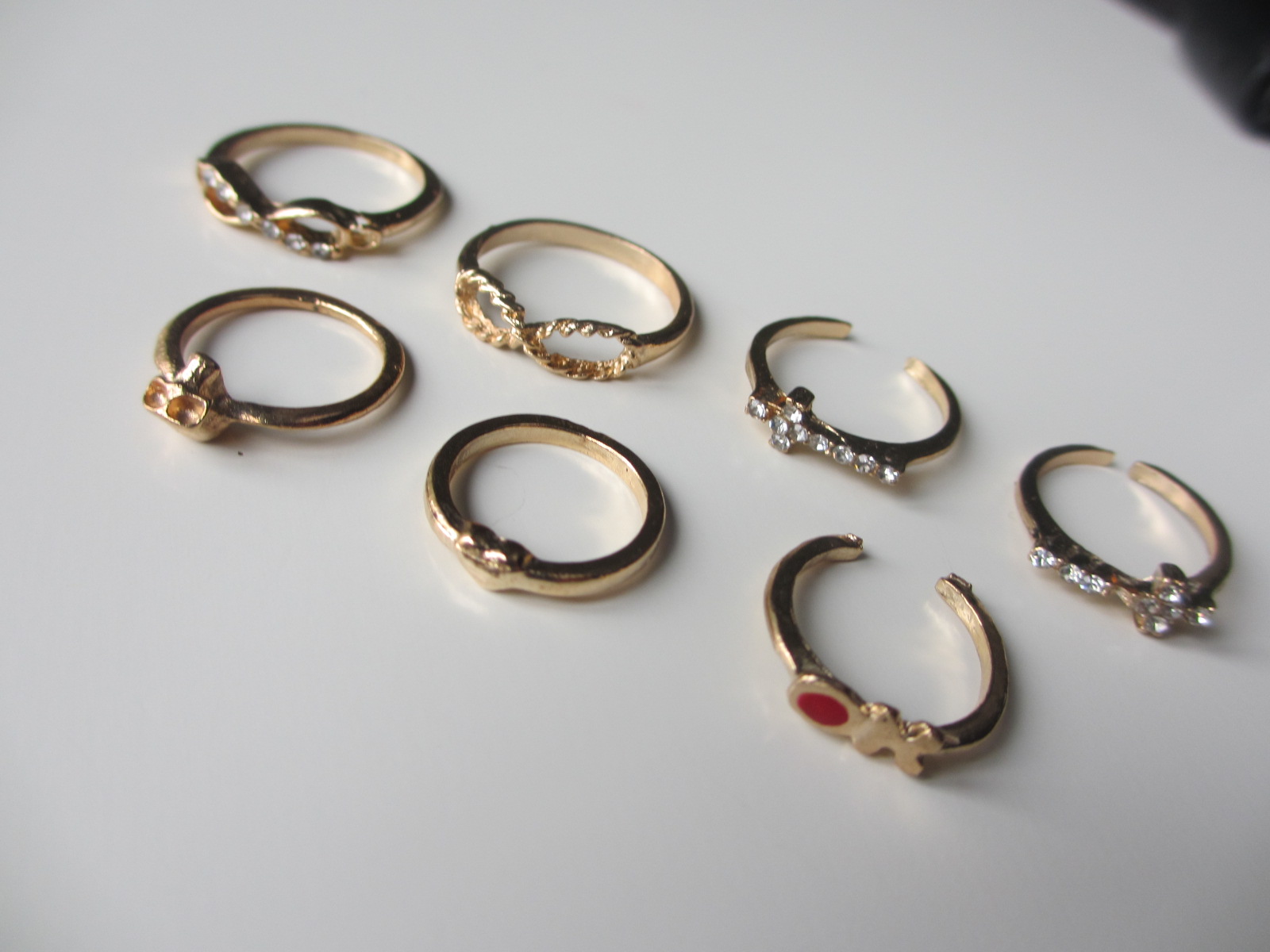This professionally taken close-up image features seven gold rings displayed on a slightly slanted white surface, indoors. The rings, which have the appearance of costume jewelry, showcase a variety of intricate designs. Two of the rings prominently feature the infinity symbol, while two others are adorned with crosses encrusted with either diamonds or rhinestones. Among the remaining rings, one has a distinct heart motif, another bears the word "OK" with the O filled in red, and one includes a gingerbread-like design element. Interestingly, four of the rings have fully closed bands, while the other three appear unfinished, with their bands not yet joined together.